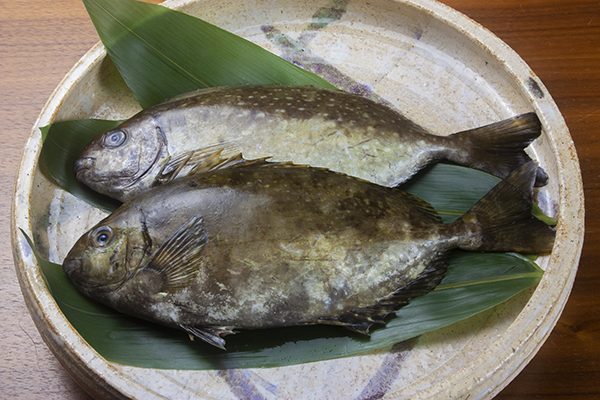In this image, we see a detailed arrangement of two whole, brownish fish, each with a dark green hue and brown spots, resting atop three vibrant green banana leaves. The fish are presented intact without any cuts or breaks. They are placed on a thick, beige-colored ceramic platter that appears to have some patterns on the inside, giving it a slightly textured look. This ceramic dish, which closely resembles clay in its composition, sits on a dark brown wooden table, unremarkable in type but providing a rustic backdrop. The overall focus of the image is clearly on the well-cooked, oval-shaped fish and their visually appealing presentation on the banana leaves within the textured ceramic platter.